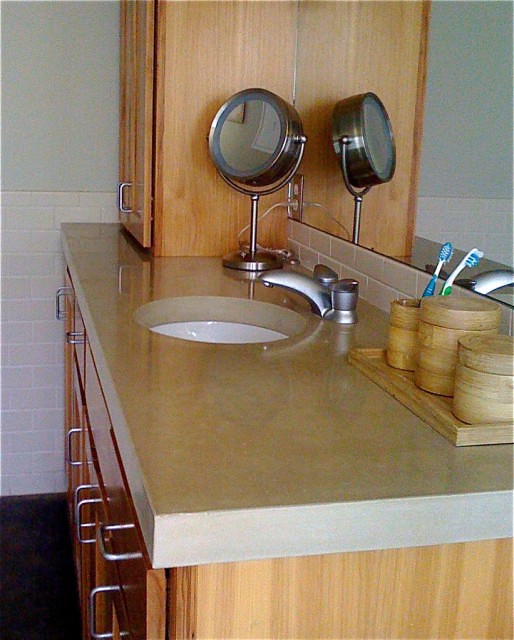This photograph showcases a bathroom vanity with a beige laminate countertop and a light tan brown wooden cabinet, embellished with simple silver-tone pull handles that resemble bent tubes. Viewed from the side, the full front of the vanity is not visible, obscuring any cabinets or drawers. On the left side of the countertop sits an additional cabinet, beside which stands a silver-tone, dual-sided mirror—one side offering magnification. A small, circular white sink occupies the center, with a matching silver-tone faucet and handles. To the right of the vanity, a tan tile backsplash extends halfway up the wall, adding a stylish touch. Completing the scene is a charming bamboo wooden tray, holding a bathroom set that includes two lidded bamboo containers and a third one holding two toothbrushes.